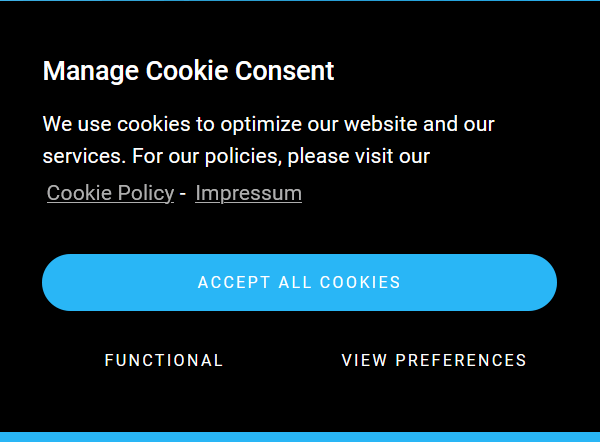The image depicts a computer or cell phone screen showing a cookie consent management prompt. The background is entirely black, resembling a black rectangle. At the top, a white text reads, "Manage Cookie Consent." Below that, a smaller white text states, "We use cookies to optimize our website and our services. For our policies please visit our," followed by grey underlined text, "Cookie Policy," indicating a clickable link. Adjacent to this, also in grey underline, is the word "Impressum," signifying another clickable link.

At the bottom of the prompt is a royal blue rectangle with rounded edges. Inside this rectangle, in bold white text, it says, "Accept All Cookies." Additionally, further down the screen, on the left in capitalized white text, it says "FUNCTIONAL," and toward the right, also in capitalized white text, it says "VIEW PREFERENCES." Both of these options are spaced apart and provide further navigation choices within the cookie consent interface. 

The overall design presents a clear and organized user interface for managing cookie preferences.